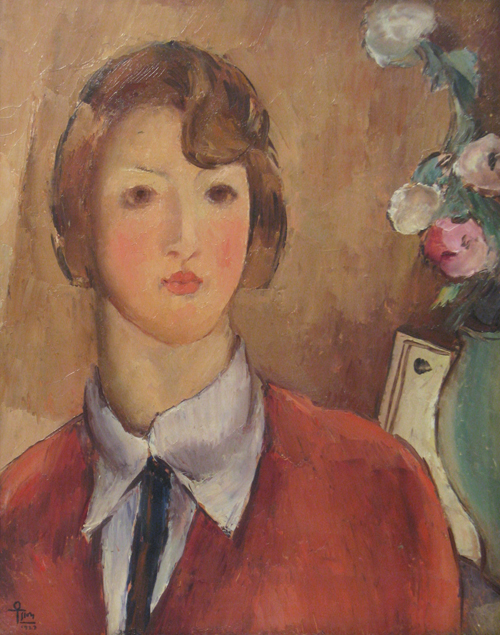This image appears to be a detailed painting of a young woman, possibly in her late teens or early twenties. She has very short, chin-length brown hair, parted to the side with a distinctive tuft sweeping towards the right side of her face. Her large brown eyes stare directly at the viewer with a serious expression, and her cheeks appear rosy, possibly due to the application of blush. She is dressed in a red sweater over a white collared shirt, which features a notably large collar and may include a thin tie, enhancing a somewhat androgynous appearance due to her thick neck. The background is a brownish wall, adding depth to the portrait. To her right, there is a teal vase filled with flowers and a corner of a book or a photo frame. The painting is signed with what could be the Egyptian Ankh symbol or a T with a circle on top, in the bottom left corner. Additionally, there is a faint indication of the numbers '1987' or '1989', suggesting that the artwork was created a few decades ago.